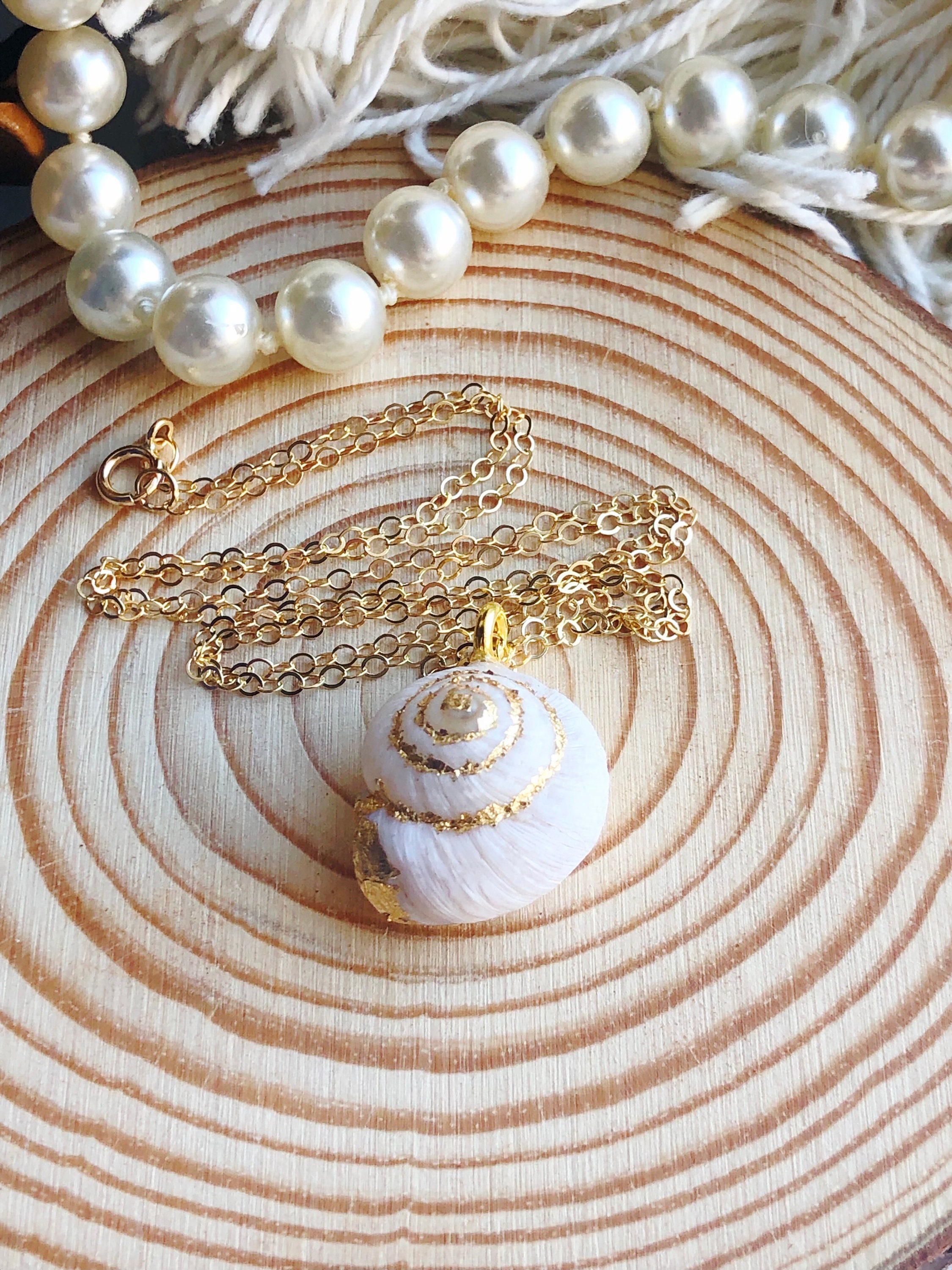The image features a detailed arrangement on a rustic wooden surface with clearly visible age rings, suggesting a tree slice. At the top of the image, white pearls strung together lie gracefully, possibly as a Christmas decoration or part of a necklace, with visible white string in between. Interspersed among the pearls are white tassels, which appear to be from a carpet or rug. Centrally placed on the wooden surface is a piece of jewelry: a delicate gold chain with a gold clasp, flowing into a white, spiral-shaped seashell pendant. The seashell, which may be manufactured rather than natural, has intricate gold glitter highlighting each curl, resembling the winding pattern of a snail's shell. The overall setting appears to be indoors.